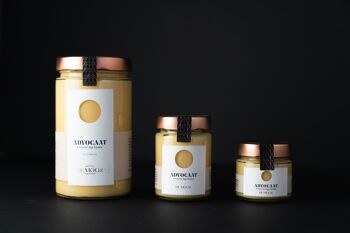This photograph features three distinct glass jars arranged from left to right against a completely black background, encompassing both the wall and the surface on which they stand. Each jar is progressively smaller in size, with the largest on the left, followed by a medium-sized jar, and the smallest on the right. The jars are filled with a creamy yellow or tan-colored substance.

All jars share similar labeling and closure features: they are topped with copper-colored lids that have a black strap or tape across the top, possibly serving as a seal. The jars have vertical white labels on the front. At the top part of each label, there is a round yellow circle, and directly below it, in black writing, is the word "ADVOCAT," spelled A-D-V-O-C-A-T (though one description mentioned variations like "A-D-V-O-C-A-A-T"). 

Around the lower section of the largest jar's label, there is another label that reads "MOOK," spelled M-O-O-K, which might be partially obscured and is not confirmed on the other jars. The jars maintain a cylindrical shape, and their size progression is approximately 8 ounces for the largest, 4 ounces for the medium, and 2-3 ounces for the smallest jar.